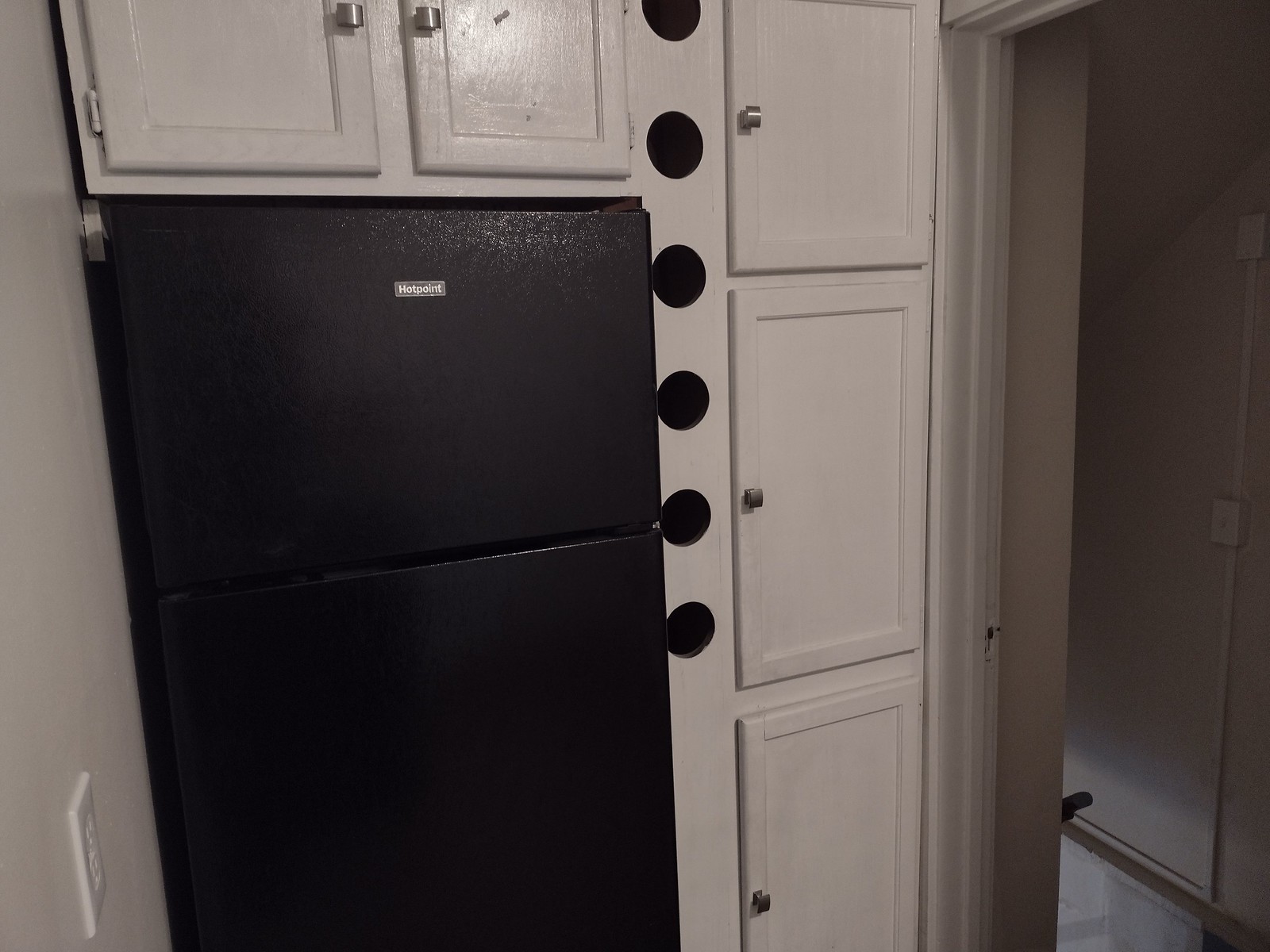This color photo showcases a kitchen centered around a black, old-fashioned Hotpoint refrigerator, featuring a top freezer and a bottom fridge. The left side of the fridge displays a white wall with an unoccupied outlet, while above the fridge, there are two white, wooden cabinet doors adorned with square silver handles. On the right side of the refrigerator is a strip of white wall decorated with six equally spaced black circles. Adjacent to this strip, three slender, rectangular white cabinets, also equipped with square silver handles, are visible. Further to the right, an open doorway reveals a glimpse of a hallway with white walls and a light-colored floor.